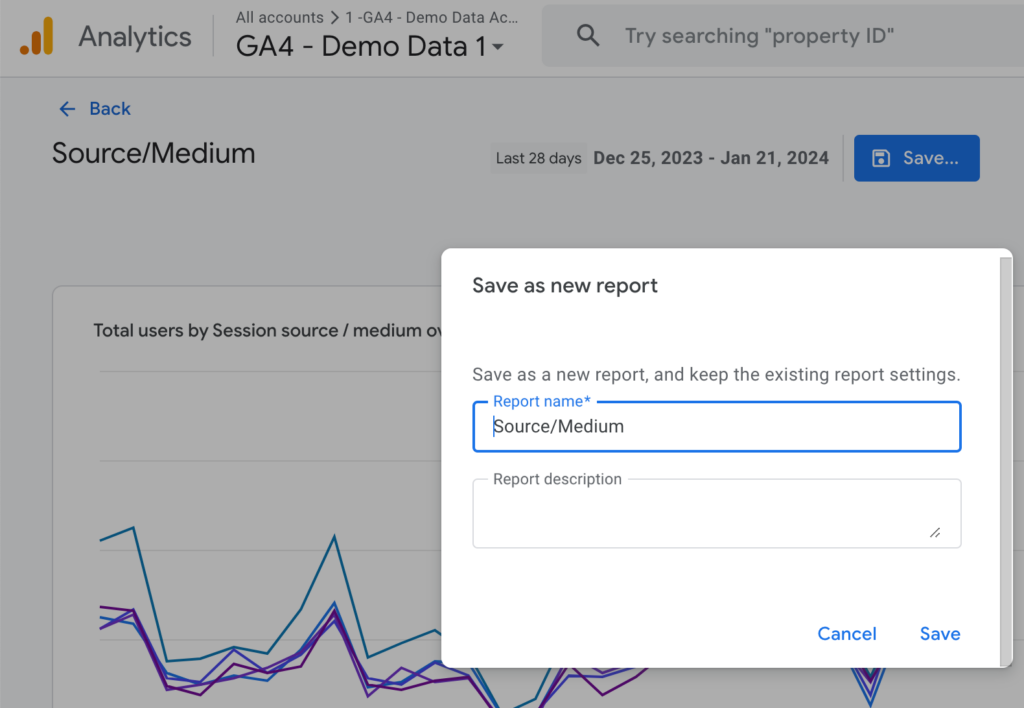The screenshot displays a section of a homepage or website, likely belonging to a company named Analytics, showcasing an Analytics report. Prominently featured is the company's logo situated on the left, comprising three bars of varying heights and shades of orange. Centrally positioned on the page is the file title, "G84 Demo Data 1," indicating the nature of the content being reviewed. Additionally, a search bar is located on the right, with the placeholder text "Try searching property ID" as an example search query.

The report in question presents data relevant to the "Source/Medium" and includes a log noting the last login period, extending from December 25th, 2023, to January 21st, 2024. To the right of the report is a button labeled "Save," used to save the demo data. Clicking this button triggers a pop-up window titled "Save as New Report." This pop-up provides a description explaining that the user can save the current settings as a new report, which entails entering a new report name (currently filled in as "Source/Medium") and optionally adding a report description (which is presently blank). The pop-up also includes options to either cancel or save the new report.

Behind the pop-up, there is a partially visible analytical graph displaying multiple lines, each distinguished by different colors, representing various data trends.